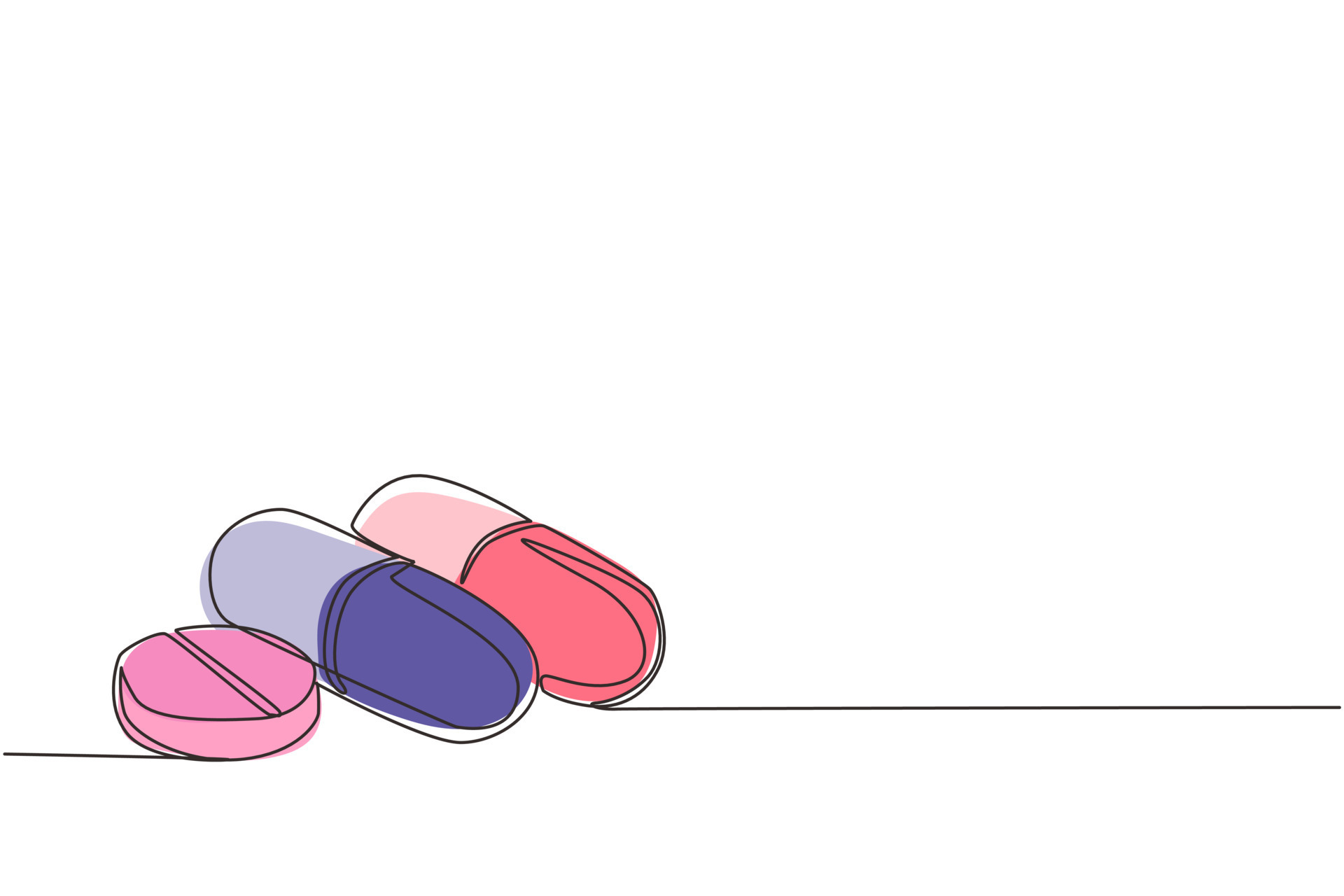The image is a simple, yet intricately drawn illustration of three pills against a white background, all outlined seamlessly by a continuous black line. Starting from the bottom left and moving to the right, the line crafts the shapes of these pills in a single, uninterrupted flow. The drawing begins with a pink round tablet positioned at a slight counterclockwise tilt, featuring a pre-scored line through its center. This tablet connects to a dual-colored capsule, with its top half in light lavender and the bottom half in a deep, dark blue. Following this, the continuous line forms another capsule, this one with a light peach upper portion and a darker pink lower portion. The line then extends to the right edge of the image. Overall, the artwork includes intricate touches like the pills' soft color transitions and neatly defined outlines, giving a sense of coherence despite the different orientations and shapes of the pills.